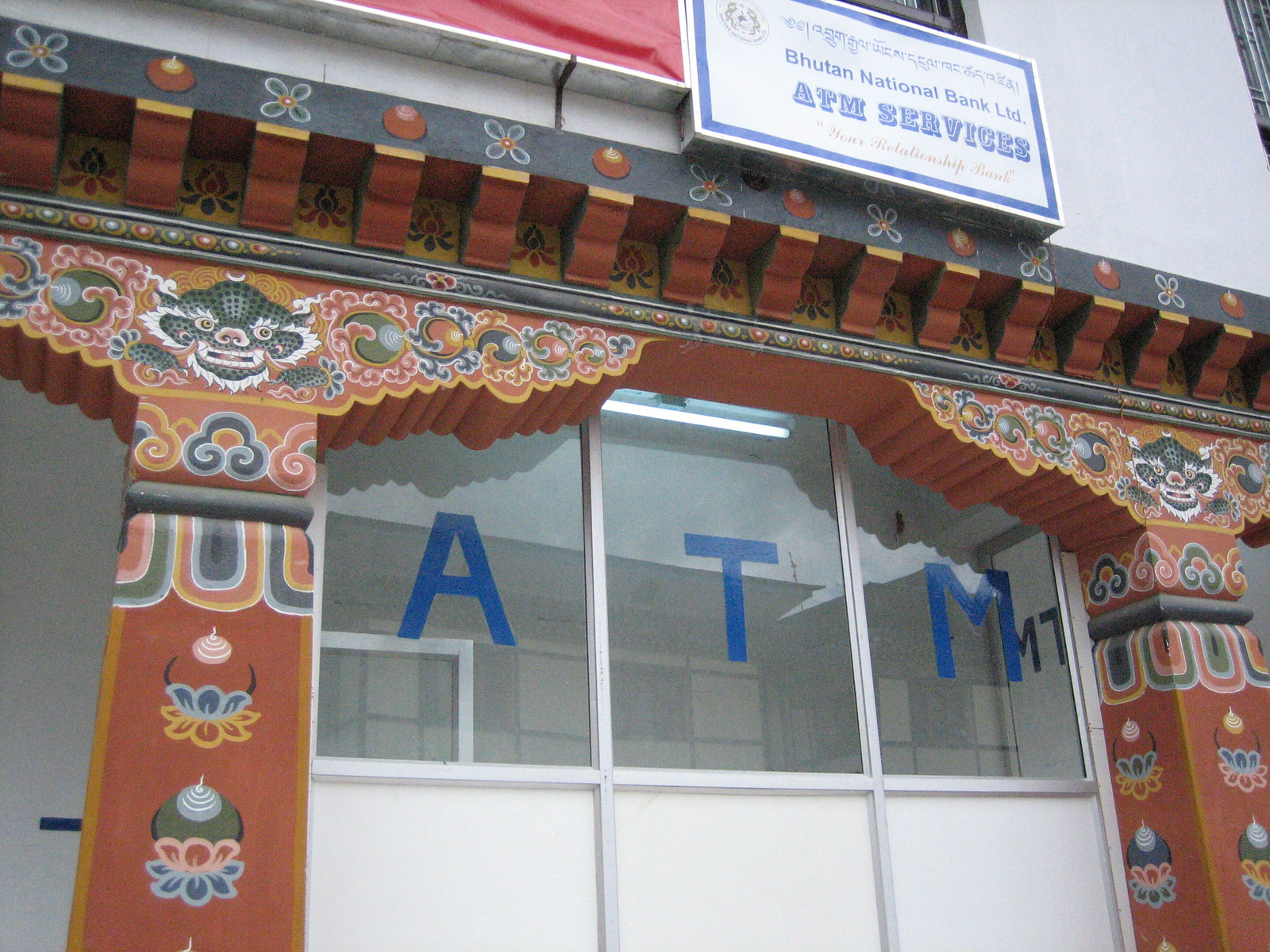The image depicts a richly decorated facade of the Bhutan National Bank LTD, with prominent ATM services. The building features elegant architectural details and is likely situated in an Asian country. At the top, a white sign with a blue rectangular border reads "Bhutan National Bank LTD" in blue text, with "ATM Services" in a thicker, larger blue font beneath it. Above the primary text, there is Middle Eastern stylized writing. In cursive, and enclosed in quotation marks below, the sign reads "your relationship bank." The building is adorned with distinctive red pillars on either side, elaborately decorated with floral and circluar patterns. Brown and green accents blend into what appears to be tribal mask features on the pillars. Reflections are visible on the windows, which display the bold, blue letters "ATM." These letters are repeated three times, each capitalized and possibly painted or affixed with stickers. Wavy designs and an apple-flower border add to the decorative appeal, framing this outdoor scene accentuated by the building's white foundation and red trim.